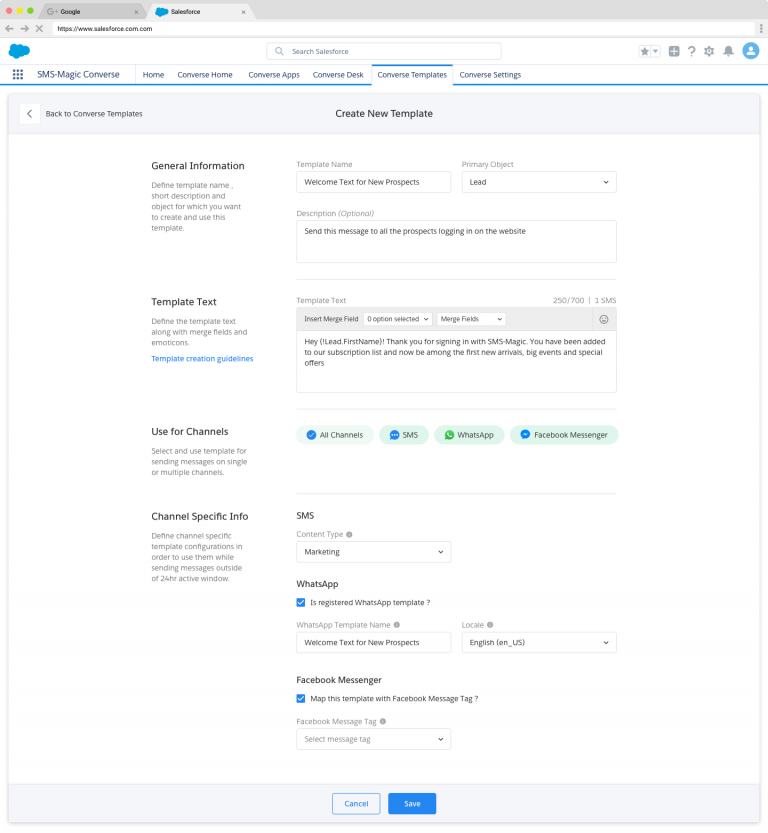This image is a detailed screenshot from a software interface, specifically Salesforce, where the Salesforce tab is active among two open tabs, the other being Google. The URL in the address bar reads 'salesforce.com', and a recognizable blue cloud Salesforce logo is displayed next to it. Below, the interface is prominently branded with "SMS-MAGIC," featuring a series of navigational options including Converse Home, Converse Apps, Converse Desk, Converse Templates, and Converse Settings. The "Converse Templates" section is currently active.

The interface content outlines steps to create a new template, organized into sections such as General Information, Template Text, Use for Channels, and Channel Specific Info. Channels listed include SMS, WhatsApp, and Facebook Messenger. Towards the bottom, there are buttons labeled 'Cancel' and 'Save' for template editing actions. In the middle of the interface, a dropdown menu allows users to select specific channels, reiterating the choices of SMS, WhatsApp, and Facebook Messenger.

Currently, the template text reads: "Hey [Lead First Name], thank you for signing in with SMS-MAGIC. You have been added to our subscription list and will now be among the first to know about new arrivals, big events, and special offers."